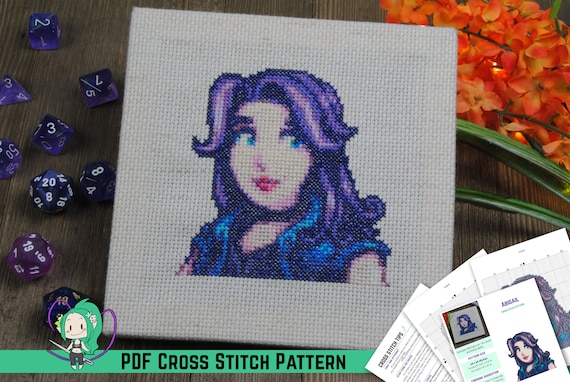This photograph captures a detailed, stitched version of Abigail from Stardew Valley, featured on a square cloth prominently placed on a wooden table. Abigail's in-game artwork is portrayed with her purple hair, blue eyes, red lips, and blue top, which is cut off at the chest, exposing her arms but not her shoulders, against a white stitched background. To the left of the image, there are several multi-sided dice, including various 20-sided and 8-sided dice, mostly purple, often used in games like Dungeons & Dragons. To the top right, an arrangement of small, fake orange flowers with long, stick-like green leaves adds a pop of color. The bottom of the image includes additional visual elements: a green-haired chibi character with text reading "PDF cross-stitch pattern" and a collection of reference sheets displaying different images of Abigail, like screenshots from various sources, as well as close-up profiles of her.